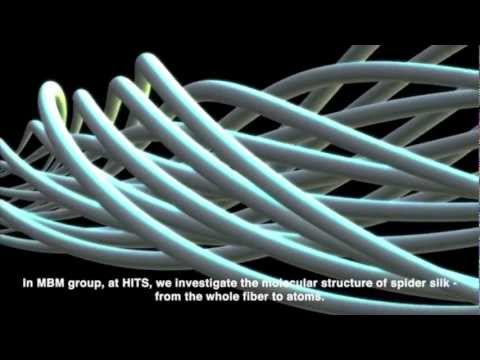The image features a detailed, close-up view of intertwined, spiraling white cylindrical structures against a solid black background. The arrangement resembles a complex web, reminiscent of the old Windows 2000 screensaver with its intricate, looping paths. The spirals and the overall composition evoke the appearance of tangled cable or hair, simulating an almost chaotic yet structured assembly. At the bottom of the image, in small white text, it reads: "In MBM group, at HITS, we investigate the molecular structure of spider silk—from the whole fiber to atoms." This text suggests that the depicted structures are an artistic representation of spider silk at a molecular level, aligning with scientific research and visualization.